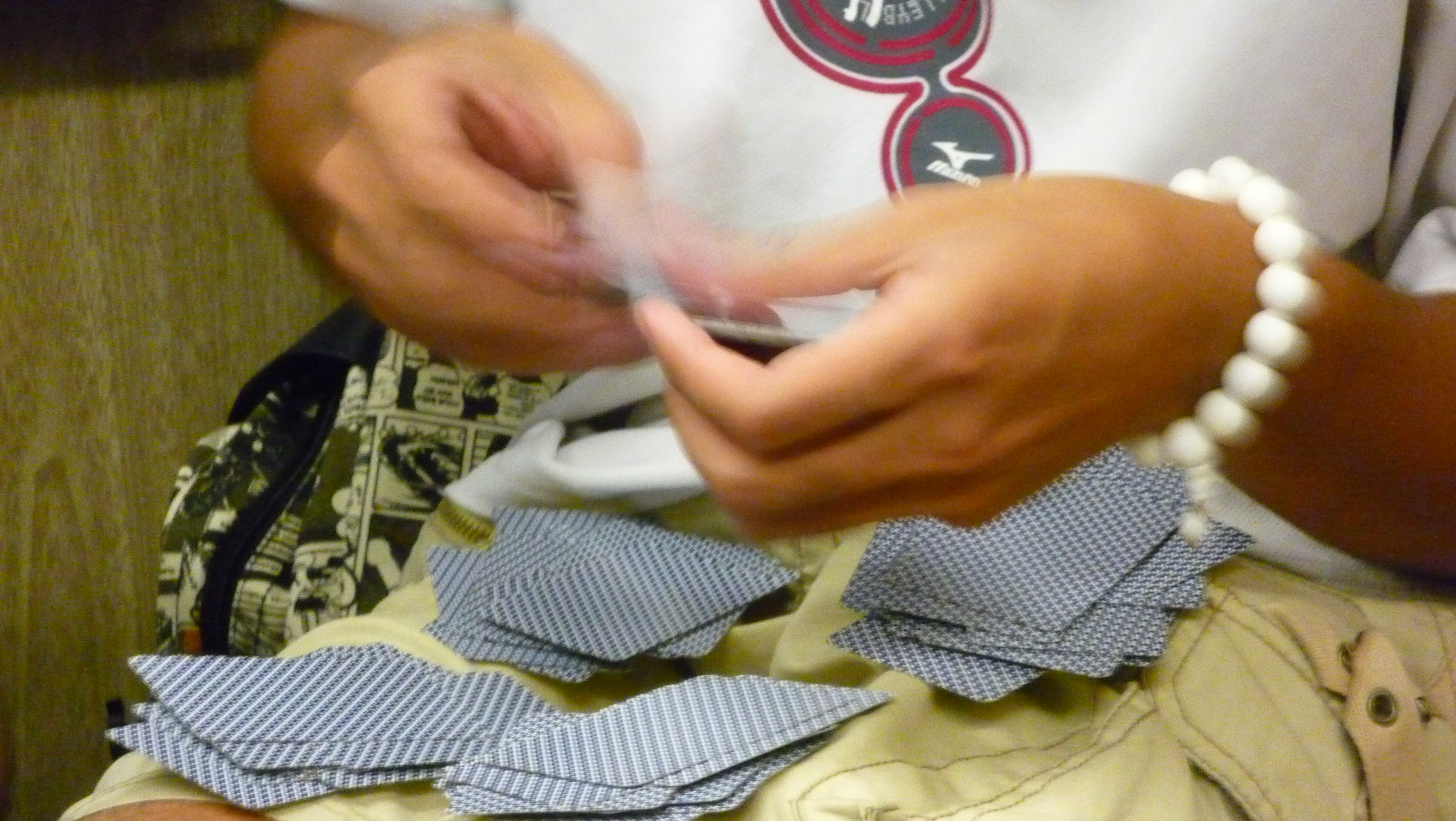In the image, a person is holding a collection of playing cards, characterized by their checkered backs. She is sorting the cards into four piles, visible on her lap and surrounding areas, though it appears she is still in the midst of doing so. The woman's hands are a blur of motion, indicating the speed of her actions. She is dressed in a white shirt adorned with a red and gray graphic that somewhat resembles a wheel, although it is not entirely clear. On her left wrist, she wears a distinctive bracelet made up of white pearls.